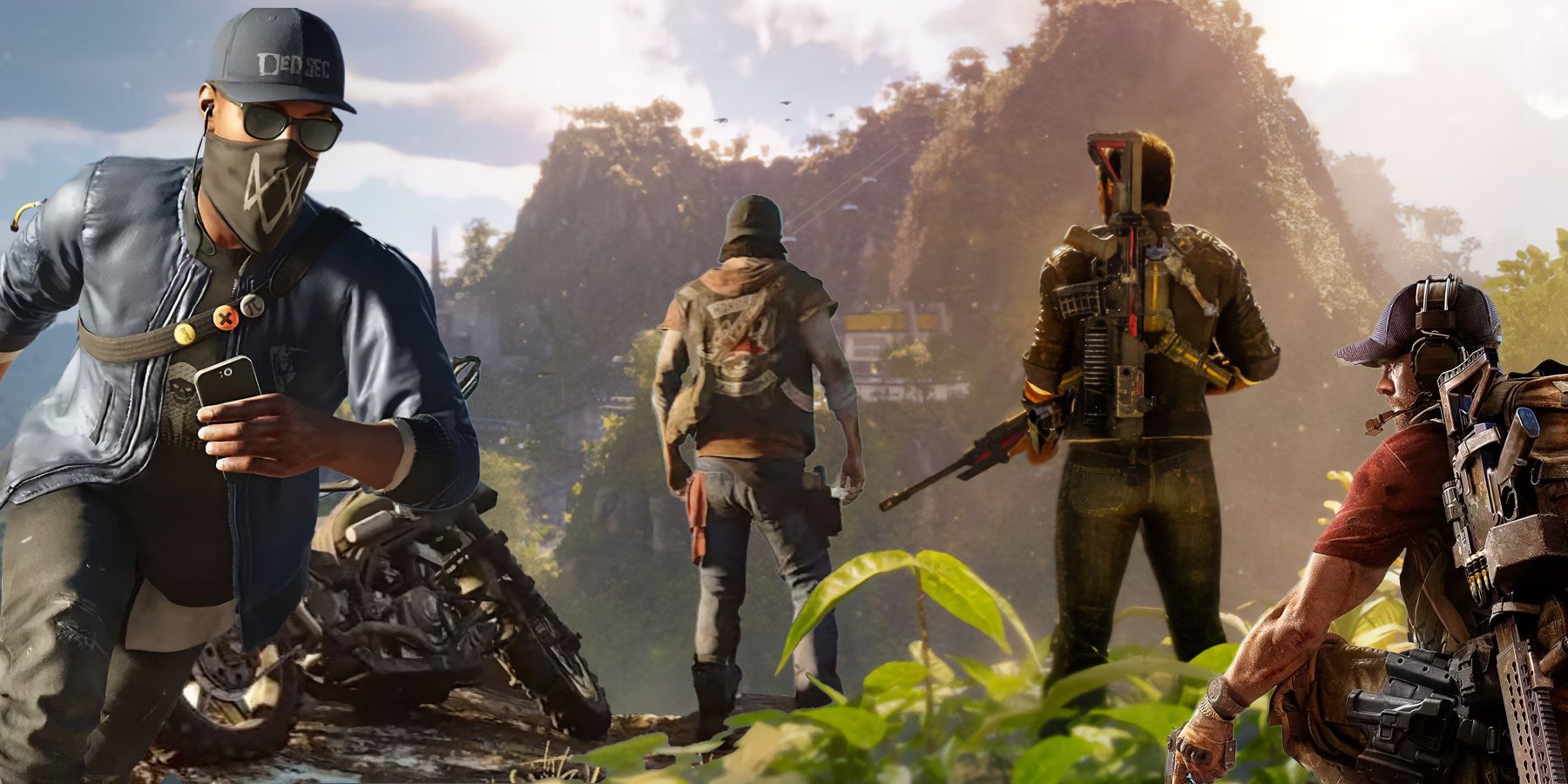In this hyper-realistic image likely from the Watch Dogs video game series, four armed men are set against a daytime mountainscape with a sky filled with dark gray clouds and rays of sunlight breaking through. The dominant palette includes browns, blues, and dark greens, emphasizing the rugged and dynamic environment.

In the foreground to the left, a man, appearing tan-skinned, is in motion, seemingly running. He dons a distinctive dark blue leather jacket and a similarly-colored DedSec hat bearing numerous pins. His face is partially obscured by a black mask and dark sunglasses. He holds a cell phone and is further equipped with a black bag strapped over his shoulder. Near him is a dark motorcycle.

At the center, two men stand with their backs to the viewer, both facing the distant mountain. They exhibit the demeanor of outlaws, each armed and wearing vests. Their poses convey readiness, contrasting with their scenic backdrop.

In the lower right corner, a muscular, dark-skinned man is kneeling. Adorned with a significant amount of weaponry, including a large rifle holstered on his back along with visible ammunition, he adds to the intense, combative atmosphere of the scene. The presence of plants and trees encircling the group, set within an Amazonian-like landscape, enhances the setting's depth and realism.